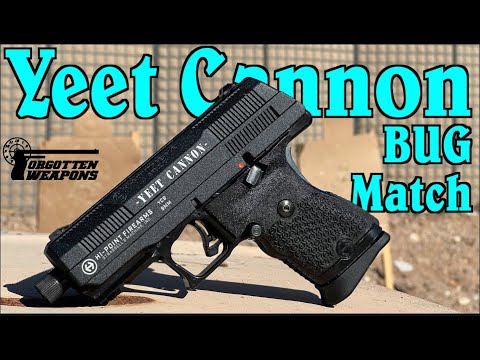A small black pistol, named the "Yeet Cannon Bug Batch," is photographed resting on a beige concrete surface. The gun is positioned at a 45-degree angle with the barrel pointing diagonally downward to the bottom left, and the handle placing it in an upside-down V shape. The short barrel of the pistol features white text, including "Yeet Cannon" and "High Point Firearm." Behind the image, the caption "Yeet Cannon Bug Batch" appears prominently in bright blue with a black outline. Additionally, a "Forgotten Weapons" logo in black is visible on the left side of the background.